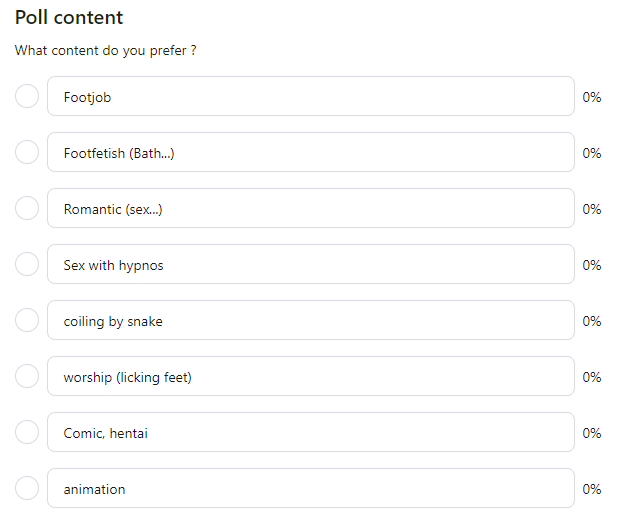In the top-left corner, there is black text that reads "Pull Content." About two inches below, the question "What content do you prefer?" is displayed. Underneath, there is a small gray circle followed by a light gray rectangular box, which resembles a search bar. Inside the box, the words "foot job" are displayed, aligned to the left, and "0%" appears to the right.

Continuing down, the text "Foot Fetish (Bath)... 0%" is listed. Below this, another line states "Romantic (Sex)... 0%". Then, the phrase "Sex with Hypnos, 0%" is mentioned, with "Hypnos" spelled out as h-y-p-n-o-s. Further down, "Coiling by Snake 0%" is indicated, followed by "Worship (Licking Feet) 0%."

Next, the text "Romantic, Hentai, 0%" is shown, with "Hentai" spelled out as h-e-n-t-a-i. Finally, at the bottom, there is a box containing the word "Animation" with "0%" to the right. This detailed list summarizes all the text and information present in the image.